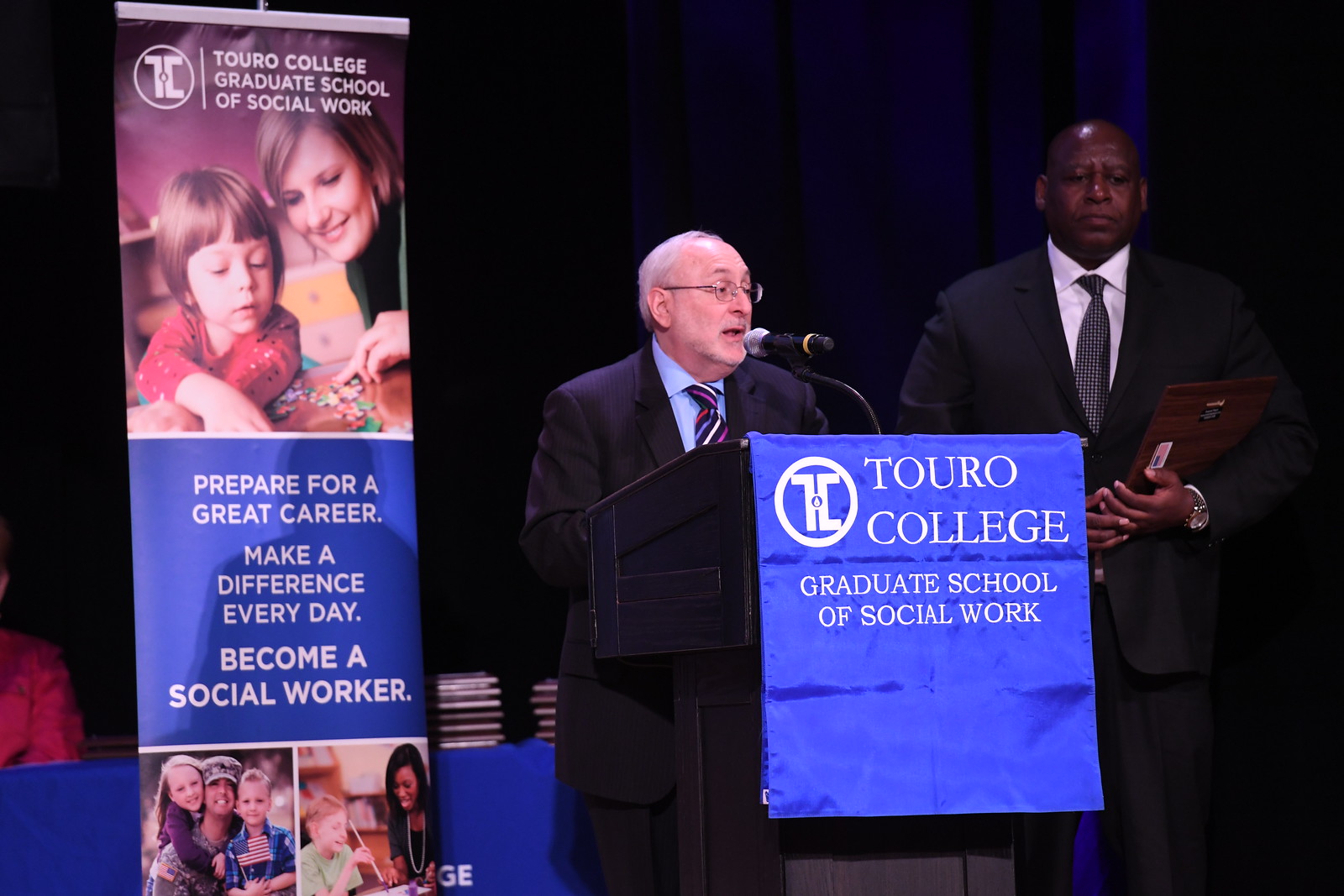In this indoor photograph, a distinguished elderly white man stands behind a black podium, speaking directly into a microphone. The podium features a blue rectangular banner with white text that reads "Touro College Graduate School of Social Work." He is dressed in a dark blue coat over a blue shirt, wearing glasses, and has sparse gray hair on his mostly bald head. To the right of the speaker (left in the image), a tall, bald black man stands quietly with a studious expression. He is attired in a black suit paired with a white shirt and a black-and-white patterned tie. He holds a brown clipboard or folder under his left arm, with his hands clasped in front of him.

Behind these individuals, a large poster displays various pictures and inviting text about social work, featuring happy people and urging viewers to "prepare for a great career, make a difference every day, become a social worker." A blue cloth-covered table in the background is adorned with books. A blue curtain stretches across the upper part of the background, flanked by darkness on either side.